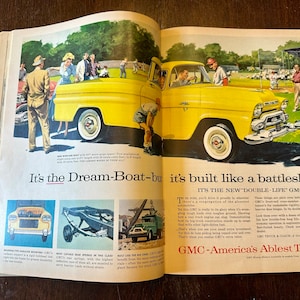The image depicts an open vintage book or magazine placed on a wooden table, showcasing a full two-page advertisement for a yellow, old-fashioned car, likely from the 1940s or 1950s. The upper half of the spread features an illustration of the car surrounded by a diverse group of onlookers, including a baseball player, a man in a suit, women in dresses, and a child inspecting the vehicle. The headline in the middle declares "It's the dream boat, built like a battleship." Below the headline, the bottom half of the left page contains three detailed blue line drawings of different parts of the car, while the right page is filled with text columns describing the car. At the very bottom of the right page, in red text, it reads "GMC, America's Ablest," though some of it is obscured. The detailed and realistic illustrations create an engaging advertisement that blends vintage charm with technical details.